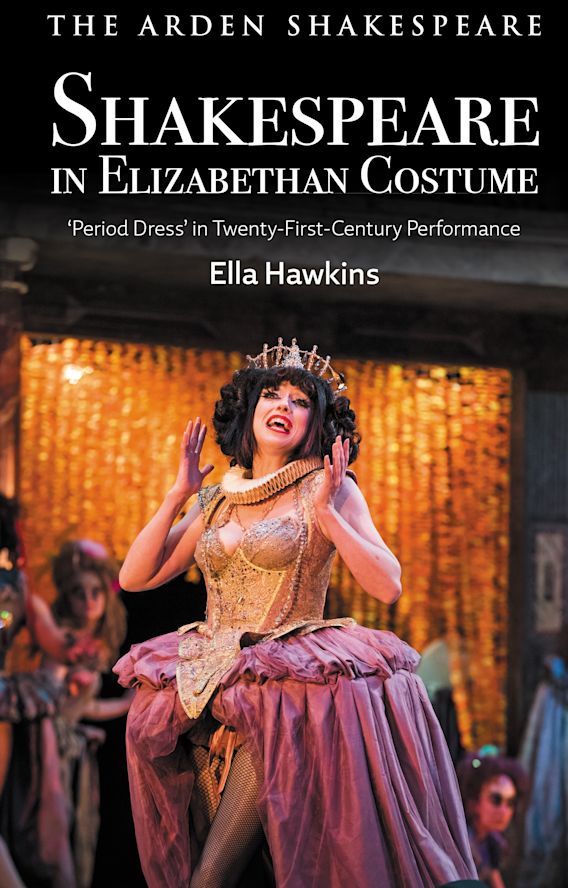The poster advertises an event titled "Shakespeare and Elizabethan Costume: Period Dress in 21st Century Performance," presented by The Arden Shakespeare. The focal point is Ella Hawkins, whose name is prominently displayed in a large sans serif font. Ella is depicted in an opulent Elizabethan-style gown, featuring a corset and large dress. The gown predominantly showcases purple, gold, and peach hues. Notable elements include a golden Shakespearean collar, similar to those depicted in portraits of Shakespeare, and an elaborate tiara adorned with golden details and possibly some gems. The composition suggests she is in the midst of a performance, evident from her expressive facial features and hand gestures. The backdrop features stage players, reinforcing the theatrical setting. The distinct fonts used for different sections of the text add to the visual appeal and highlight the key aspects of the performance.